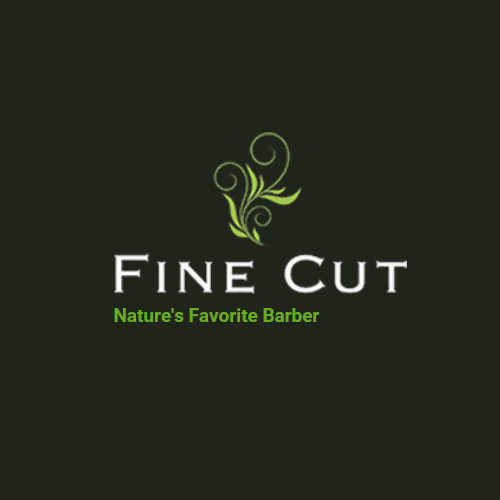The image features a dark, almost black, background with a centered logo composed of text and a decorative accent. At the top of the image, there is a light green, intricate vine design with three curled stems and seven long leaves. Below this decorative element, the text "Fine Cut" is prominently displayed in bold, white, capital letters. Directly beneath "Fine Cut," in smaller neon green letters, it reads "Nature's Favorite Barber," with capitalized N, F, and B. The logo, likely intended for a company, is symmetrically arranged and appears professionally designed, possibly for use on business cards or a company website. The color palette includes shades of green, white, and black, giving it a sleek and nature-inspired aesthetic.